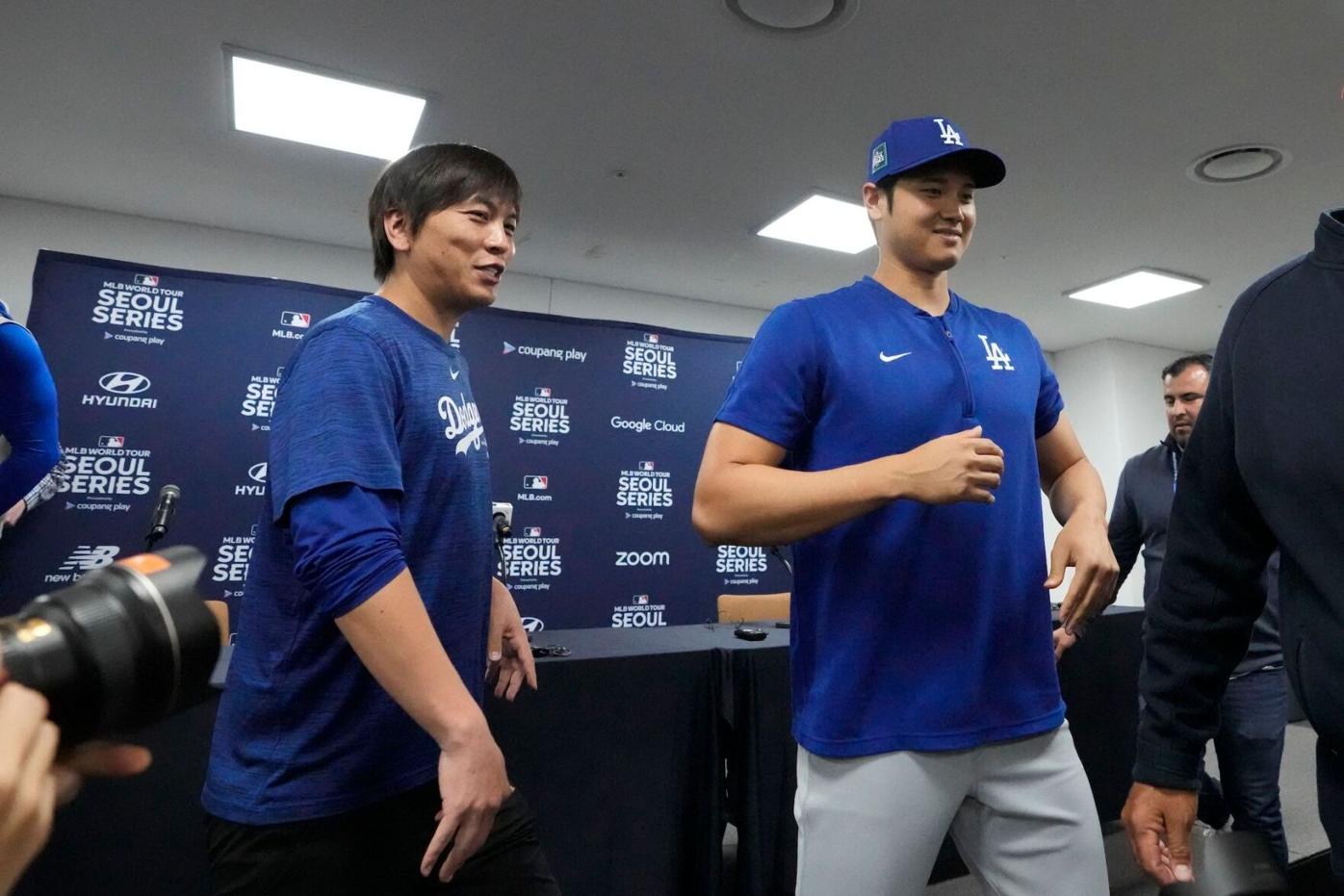This detailed, color photograph captures a moment indoors featuring the famous L.A. Dodgers baseball player Shohei Ohtani and his translator. The image is taken from a lower angled view, focusing prominently on the two men. Shohei Ohtani, positioned on the right, is dressed in a blue L.A. Dodgers T-shirt featuring both a Nike logo and the LA emblem, white pants, and a blue Dodgers hat. His translator stands to his left, an Asian man with short hair, dressed in a long-sleeved Dodgers shirt pushed up to the elbow. Both men are looking towards the right, sharing a smile.

In the left corner of the photo, you can glimpse a black long lens of a camera being held by someone capturing the scene. The background is adorned with a backdrop indicating "Seals Soul Series," along with the MLB and Hyundai logos, hinting at a major league baseball event possibly related to South Korea. Additional figures are partially visible on the far right, with one person's face partly shown and another in a dark shirt showing only a small part of their body. The setting appears to be post-Q&A, evident by a tabletop with a dark blue sheet seen behind them. This image encapsulates the camaraderie between Shohei Ohtani and his translator amid a professional backdrop.